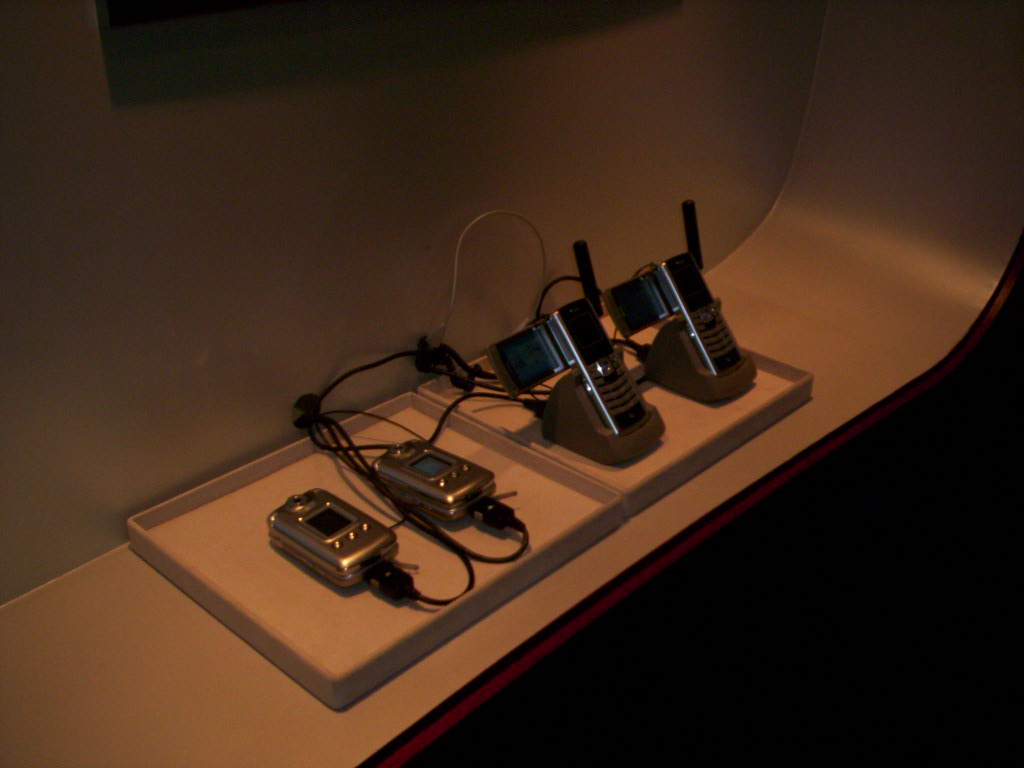The image shows a dimly lit indoor scene with a brownish tint, possibly of a small desk or bench area, likely in a hotel room. The bench extends from the left corner of the room and curves upward at the right end, attaching to the wall both at the top and bottom, and it is covered in gray laminate. Two rounded-edge white trays are placed on this surface, bordered by a thin red line along the edge.

In the left tray, there are two silver flip phones lying side by side. Each phone is connected to a black charging cable, with the cords plugged into the bottom of the phones. These phones have tiny screens and three buttons below the screens. 

In the tray on the right, two plug-in style landline phones, reminiscent of early Motorola models, are positioned in their charging cradles. These phones feature small antennas on the side, display screens extending from the left, and silver buttons with black tops. 

A soft white light illuminates the desk area, highlighting the charging phones. Behind the shelf, the wall is painted gray. Above the shelf, part of a larger, possibly rectangular item (a TV or picture frame) is partially visible extending off the top of the image.